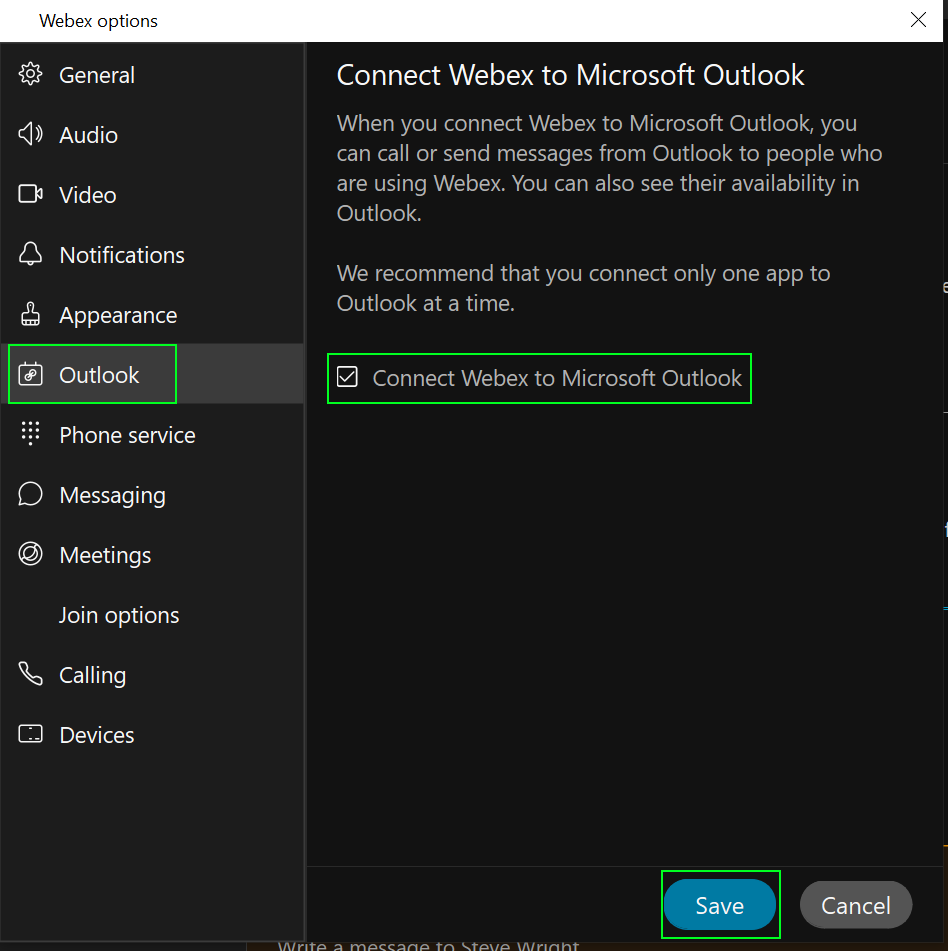This image is a screenshot of the settings section in the Webex application. The background is black with a vertical grey line that splits the image down the left side, occupying about one-third of the space. On the left side of the grey line, there are navigational tabs listed vertically, including "General," "Audio," "Video," "Notifications," "Appearance," and "Outlook." The "Outlook" tab is highlighted with a green box.

To the right of this menu, the main content of the screen is displayed. At the top right, there is an instruction: "Connect Webex to Microsoft Outlook." The option "Connect Webex to Microsoft Outlook" is also checked, indicated by a green-highlighted box with a checked white checkbox inside.

Additionally, a descriptive text below the main instruction reads: "When you connect Webex to Microsoft Outlook, you can call or send messages from Outlook to people who are using Webex. You can also see their availability in Outlook. We recommend that you connect only one app to Outlook at a time."

On the bottom right of the screen, there are two buttons. The "Save" button is highlighted in a green box, and next to it is the "Cancel" button.

Overall, this image illustrates the integrated settings options between Webex and Microsoft Outlook, emphasizing the connectivity and usage recommendations.